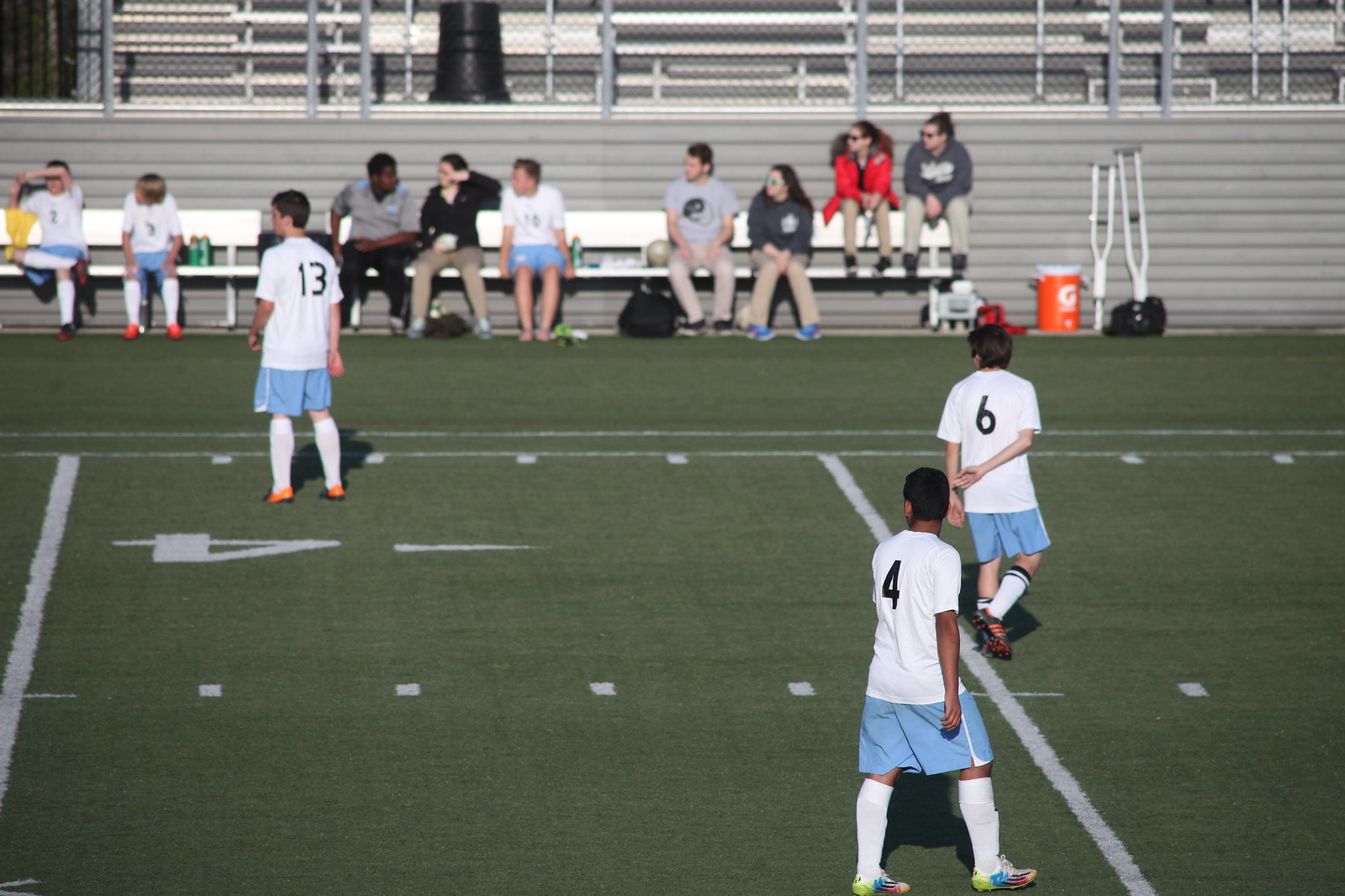The image captures a soccer match in progress on a green football field decorated with white lines. There are three teenage boys in the foreground, each wearing white jerseys with black numbers, baby blue shorts, and white socks. One of the boys sports the number 13, another has the number 6, and the third is number 4. The scene is set during the daytime, giving clear visibility of the action and surroundings. 

To the right, a Gatorade cooler and a pair of gray crutches are positioned near a metal bench. In the background, a small audience is gathered on metal bleachers, comprised of both players in uniforms and spectators in casual clothing, engaged in conversation while observing the game. The field itself appears to be artificial turf, indicating a well-maintained surface suitable for multiple sports. The overall atmosphere captures the energy and casual social environment typical of youth sports events.